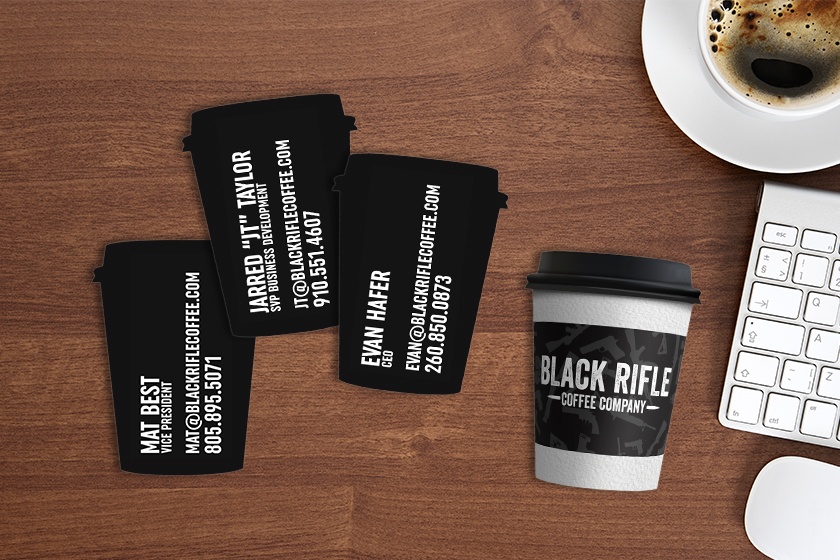This image showcases a unique 2D display of items that appear to be business cards designed in the shape of coffee mugs, each containing detailed information such as names, job positions, emails, and possibly phone numbers. Three of these mug-shaped cards are prominently displayed, suggesting they are intended for distribution. Adjacent to these cards is a physical coffee mug emblazoned with the logo of "Black Rifle Coffee Company," indicating a coffee shop setting. Additionally, a steaming cup of coffee is positioned at the top right corner of the image, enhancing the coffee-themed ambiance. A keyboard is visible in the background, and a computer mouse is partially seen in the bottom right corner, hinting at a desk setup. The image seems to be a carefully curated template rather than a real-life scene.